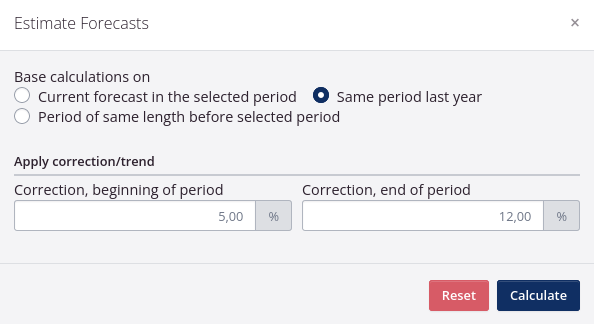This image is a screenshot of a website window, featuring a clean and structured layout primarily utilized for estimate forecasts. At the top, a white header with thin gray text on the left reads "Estimate Forecasts." On the far right of this header, there is a small gray "X" icon for closing the window.

The main body of the website has a light gray background. In the upper left corner, small text reads "Base Calculation On." Directly beneath this text, three radio buttons are displayed. The two radio buttons on the left are white circles with medium gray outlines, indicating they are not selected. The first button is labeled "Current Forecast in the Selected Period," and the second button is labeled "Period of Same Length Before Selected Period." The third radio button, located to the right of the first two buttons, is marked by a filled-in dark blue circle, indicating it is selected. The text next to this button reads "Same Period Last Year."

Below this section, the text "Apply Correction / Trend" is written in bold on the left. Beneath this bold text, there is a moderately thick medium gray line dividing the sections. Under this line, there are two text boxes. 

The first text box, positioned on the left, has a white background and displays the value "5,00." Next to it, on the right, is a medium gray box containing a dark gray percentage sign (%). This section is labeled "Correction Beginning of Period" above the text box.

The second text box, situated to the right of the first, follows a similar layout but is labeled "Correction End of Period" above it. The number inside this box is "12,00."